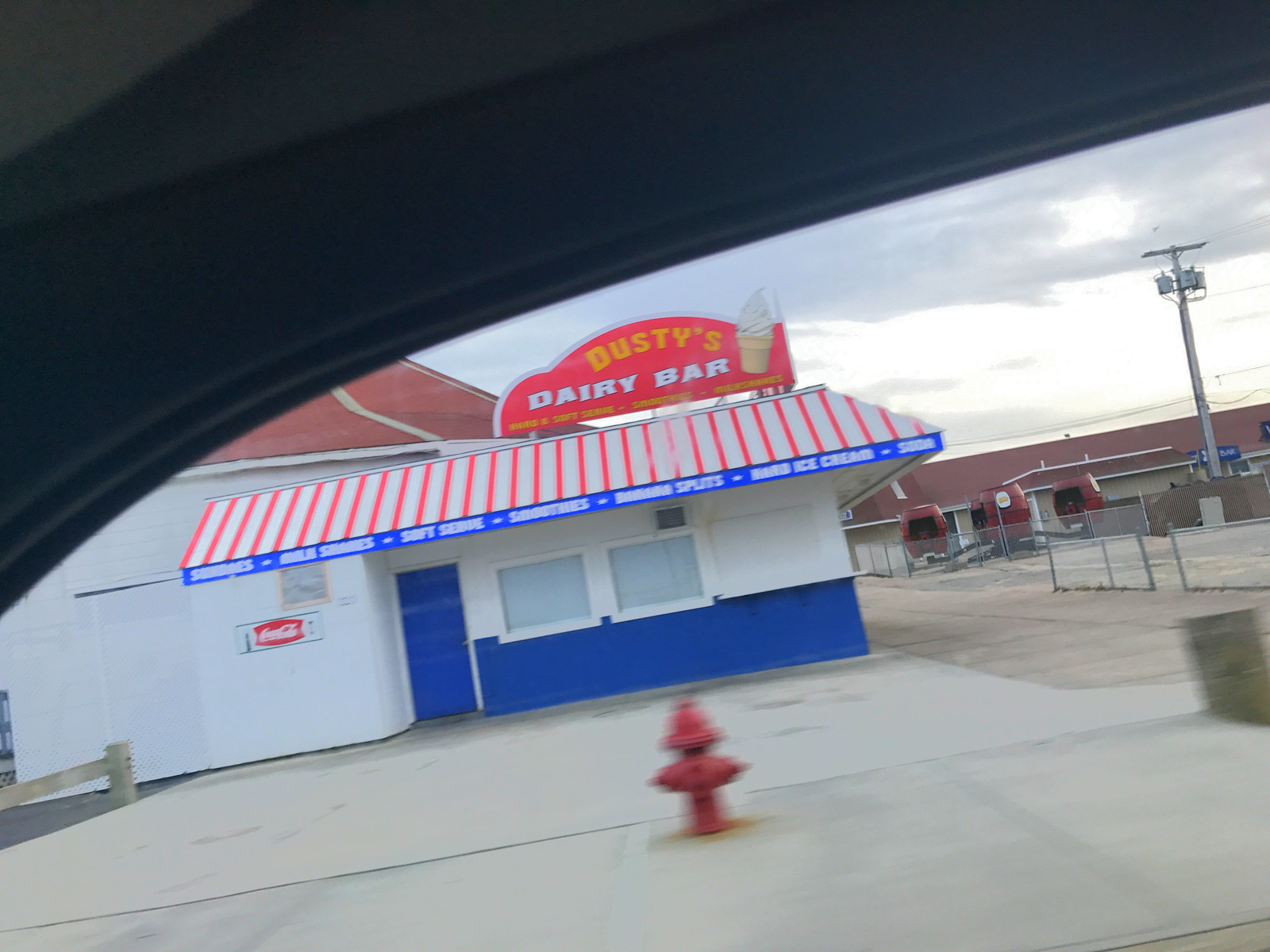Captured from the passenger seat of a car, this image features a small shop with large outdoor windows. The shop, named "Dusty's Dairy Bar," is clearly identified by a sign adorned with a swirl-topped ice cream cone. The establishment is characterized by its red and white awning, which is complemented by a blue trim at the bottom. Prominent on the storefront are the words "Ice Cream" and "Soft Serve," though other details are less discernible. In the foreground, a red fire hydrant slightly out of focus stands sentinel. To the right, a whimsical carnival ride resembling teacups but styled as apples adds a playful touch to the scene, suggesting a setting filled with community charm and leisure activities.